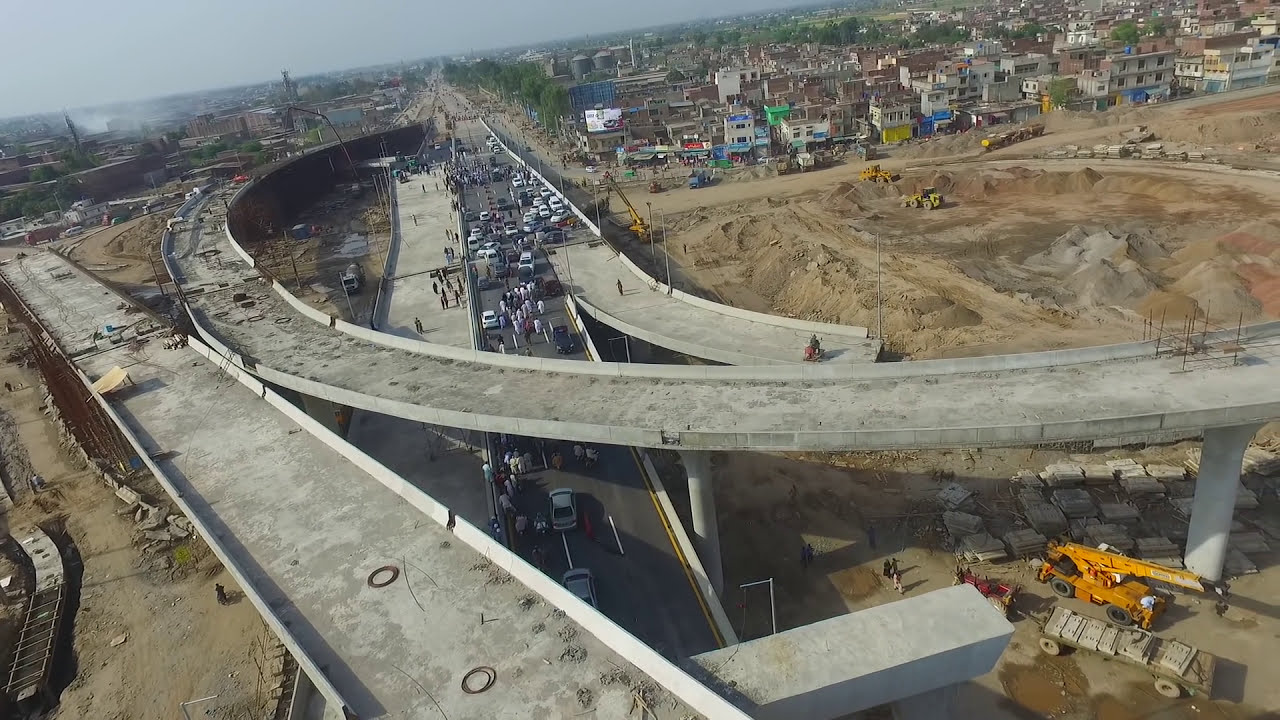This detailed aerial photograph captures a horizontally aligned, rectangular scene of a freeway under construction. The image is taken during the day under a cloudless sky. In the upper right-hand corner, there is a cluster of indistinct buildings, likely apartment complexes. As you move towards the center on the right side, there is a large dirt area with yellow construction vehicles, indicating the construction of a new overpass. One of these curved overpasses stretches from the middle right across to the upper left, still under construction with no vehicles on it. Beneath it, another partially built overpass is visible, with some people walking on it. In the lower left-hand corner, another under-construction road runs from the top to the middle of the image, supported by pylons and surrounded by dirt. The main road, filled with cars and numerous pedestrians, runs across the center at an angle. Additional details include a yellow crane in the bottom right corner and the presence of various colors like gray, brown, yellow, blue, green, black, and white, reflecting the diversity of construction materials and surroundings.